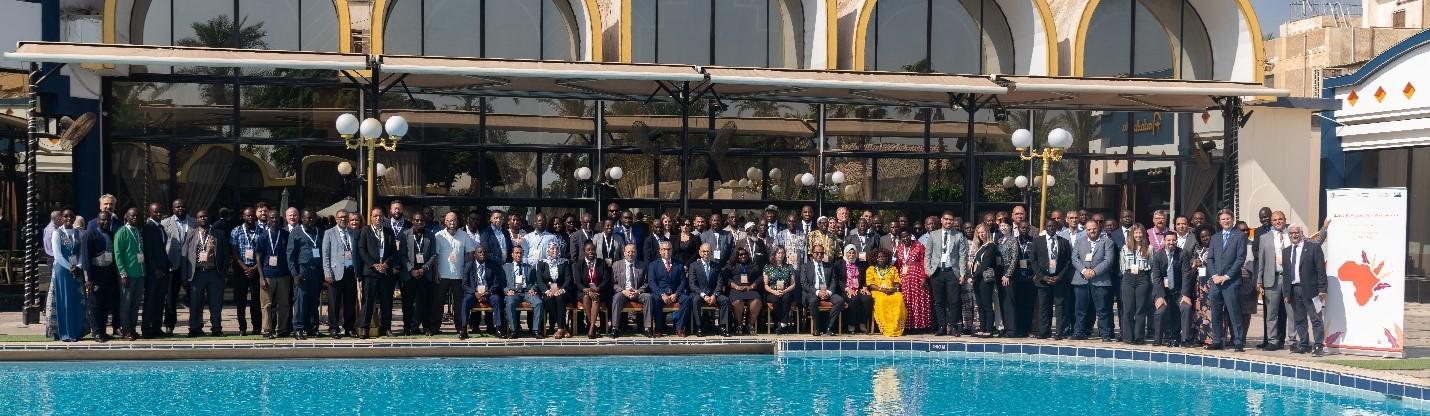The image captures a large group of people, likely numbering over 100, gathered around the edge of an Olympic-sized swimming pool. The pool, featuring blue tiles and crystal-clear water, occupies the foreground. Most of the attendees are dressed in business suits and dresses, indicating a formal occasion. A row of people is seated on chairs near the center, while the remainder stand behind them, extending to both sides. Situated prominently on the right side of the image is a tall white rectangular banner displaying a red map of Africa. In the background stands a striking white building with semicircular, arch-shaped windows that incorporate yellow triangles and slats. The building, accented with blue along the edges, also features some glass elements. Illuminating the scene are several high-standing lamps with gray bulbs. The overall setting is bright and sunny, enhancing the vibrant and formal atmosphere of the gathering.